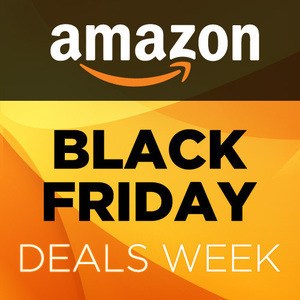The image features a striking Amazon advertisement set against a black square backdrop. The top third of the image is dominated by a dark brown section adorned with the white Amazon logo and its distinctive orange arrow underneath. The remaining two-thirds are awash with a gradient of orange and yellow hues. It starts with a deeper orange in the bottom left corner, transitions to a brighter yellow towards the center, and circles back to a richer orange at the top right edge. 

At the center of this gradient is the bold and capitalized text "BLACK FRIDAY" in black, immediately grabbing attention due to its stark contrast against the vibrant background. Beneath "BLACK FRIDAY," in a finer, smaller font, is the phrase "Deals Week," which, while noticeable, takes a backseat to the primary message. The overall design ensures that the viewer's focus is first drawn to the Amazon branding and then irresistibly towards the announcement of Black Friday deals.